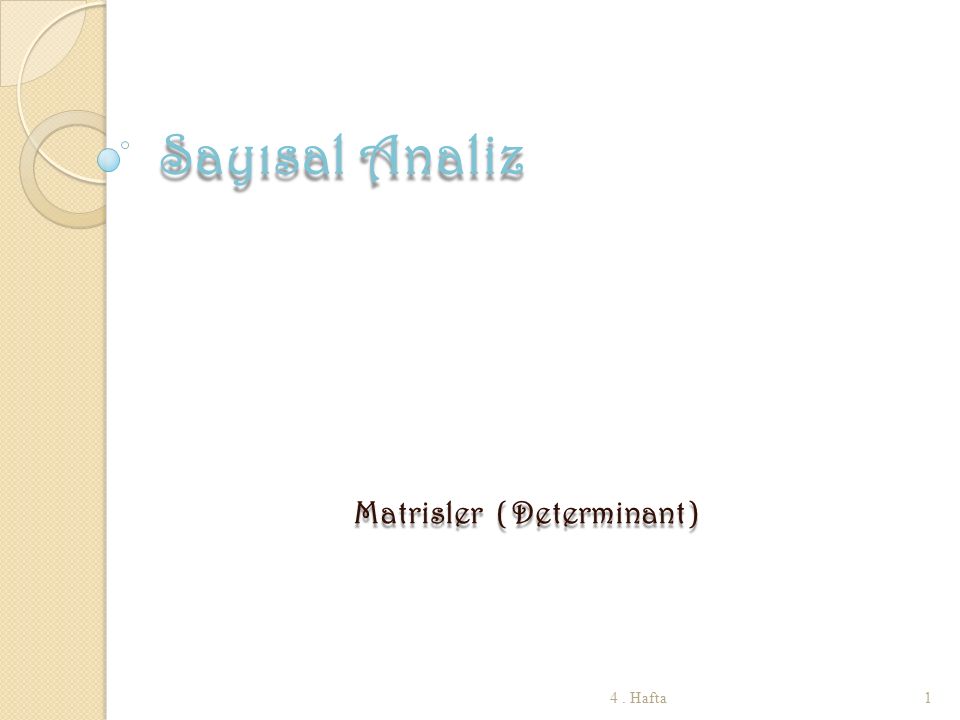The square image, with a very faint visible border at the bottom, appears to resemble the cover of a book or brochure, set on a completely white background. On the left side of the image, there is a vertically aligned tan-colored strip, extending the full height of the image. Towards the top of this strip, there are multi-colored white and beige circles, adding intricate details against the tan backdrop. Adjacent to this strip is a tiny turquoise dot. 

To the right of the tan strip is prominently displayed text in a fancy blue font with a gray shadow effect, spelling out "SAYISAL FINALIZ." Below this blue text, in smaller black letters, there is the phrase "matrisler (determinant)." Further down, at the bottom of the image, finely printed black text reads "For Hafta," and in the bottom right corner sits a standalone number "1." The overall composition combines detailed elements and varied typography, giving it a polished, meticulous appearance.